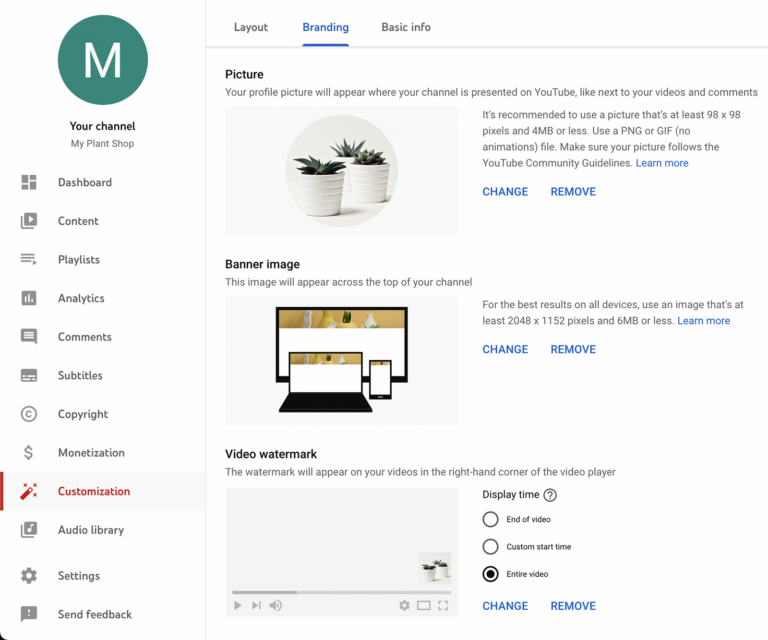This image appears to be a detailed screenshot from a YouTube channel's customization settings. The interface is displayed against a white background with gray font.

In the top left corner, there is a green circle with a white letter "M" which might be the profile icon. Below this icon, there is text reading "Your channel" followed by "My Plant Shop," presumably the name of the channel.

On the left-hand side, a vertical menu lists various navigation options, each accompanied by a relevant icon. The options include Dashboard, Content, Playlists, Analytics, Comments, Subtitles, Copyright, Monetization, Customization, Audio Library, Settings, and Send Feedback. The Customization tab is selected and highlighted in light gray with red font. Its icon is a small magic wand with three stars around it.

On the right-hand side, the options are related to channel branding, organized under tabs: Layout, Branding, and Basic Info. The Branding tab is selected, indicated by blue underlined text.

There are three sections under Branding:

1. **Picture:**
   - Information indicates that the profile picture will appear next to the channel's videos and comments.
   - Recommendations suggest using an image that is at least 98 by 98 pixels and 4 MB or less, in PNG or GIF format (no animations), and compliant with YouTube Community Guidelines.
   - Below this, there are "Change" and "Remove" buttons.
   - An image of the current display picture shows three plants in white pots.

2. **Banner Image:**
   - Describes that the banner image will appear across the top of the channel page.
   - For optimal display across all devices, an image of at least 2048 by 1152 pixels and 6 MB or less is recommended.
   - Buttons for "Change" and "Remove" are available.
   - The current banner image, seen beside a mock-up on various devices (screen, laptop, and phone), is yellow and features more plants in pots.

3. **Video Watermark:**
   - Explains that the watermark will appear at the bottom right corner of the video player.
   - There are options to display the watermark at the end of the video, from a custom start time, or throughout the entire video. The "entire video" option is selected.
   - "Change" and "Remove" options are present.
   - A mock-up shows the display picture positioned in the bottom right corner of a blank video screen.

Overall, the screenshot captures the detailed settings and customization features available for a YouTube channel, focusing on branding elements such as the profile picture, banner image, and video watermark.